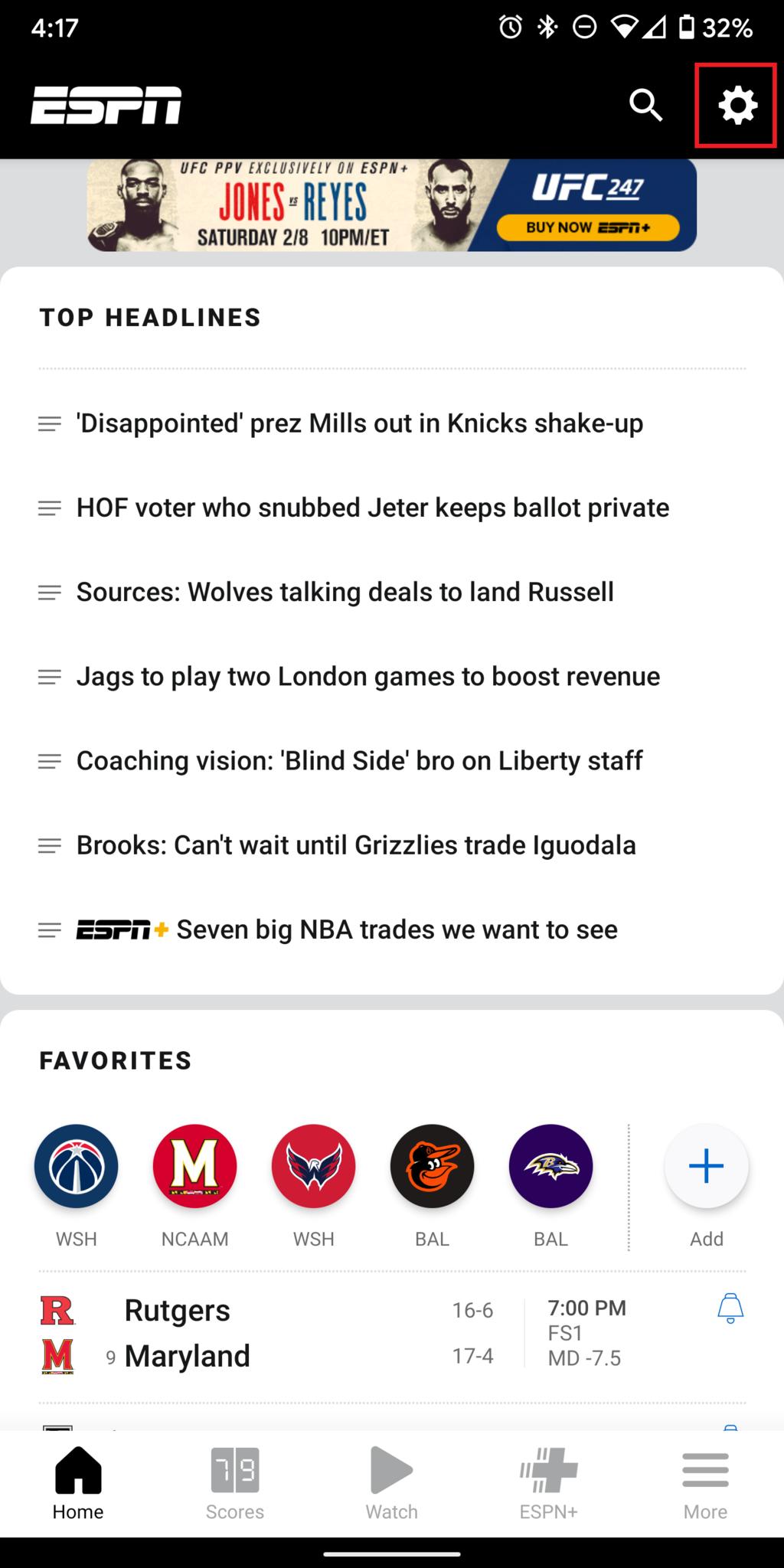This image is a cropped mobile screenshot from the ESPN app. In the top left corner, the recognizable white ESPN logo is prominently displayed. Adjacent to the logo, on the right, there is a search icon followed by a cogwheel icon, which is emphasized with an edited red box to draw attention to it.

Directly beneath this, there is a banner advertisement for UFC 247. The left side of the banner shows the event promotional graphic, while the right side features the text: "UFC 247 buy now on ESPN plus."

The main body of the page has a clean white background. At the top left, the section title "Top Headlines" is bolded. The vertical list of headlines includes the following: 
1. "Disappointed Prez Mills out in Knicks shakeup.”
2. "HOF voter who snubbed Jeter keeps ballot private."

At the bottom of the screenshot, there's a white box labeled "Favorites." Inside, a horizontal line of circular team logos is displayed, representing the user's favorite teams. At the far right of this line is a circle with a blue plus sign, labeled "Add" in small grey letters, indicating an option to add more favorite teams.

Just below the "Favorites" section, the score listing for the Rutgers vs. Maryland game is shown. The names of the teams are on the left, followed by their records. To the far right, the scheduled start time of the game is displayed, along with the broadcasting channel and an alert icon.